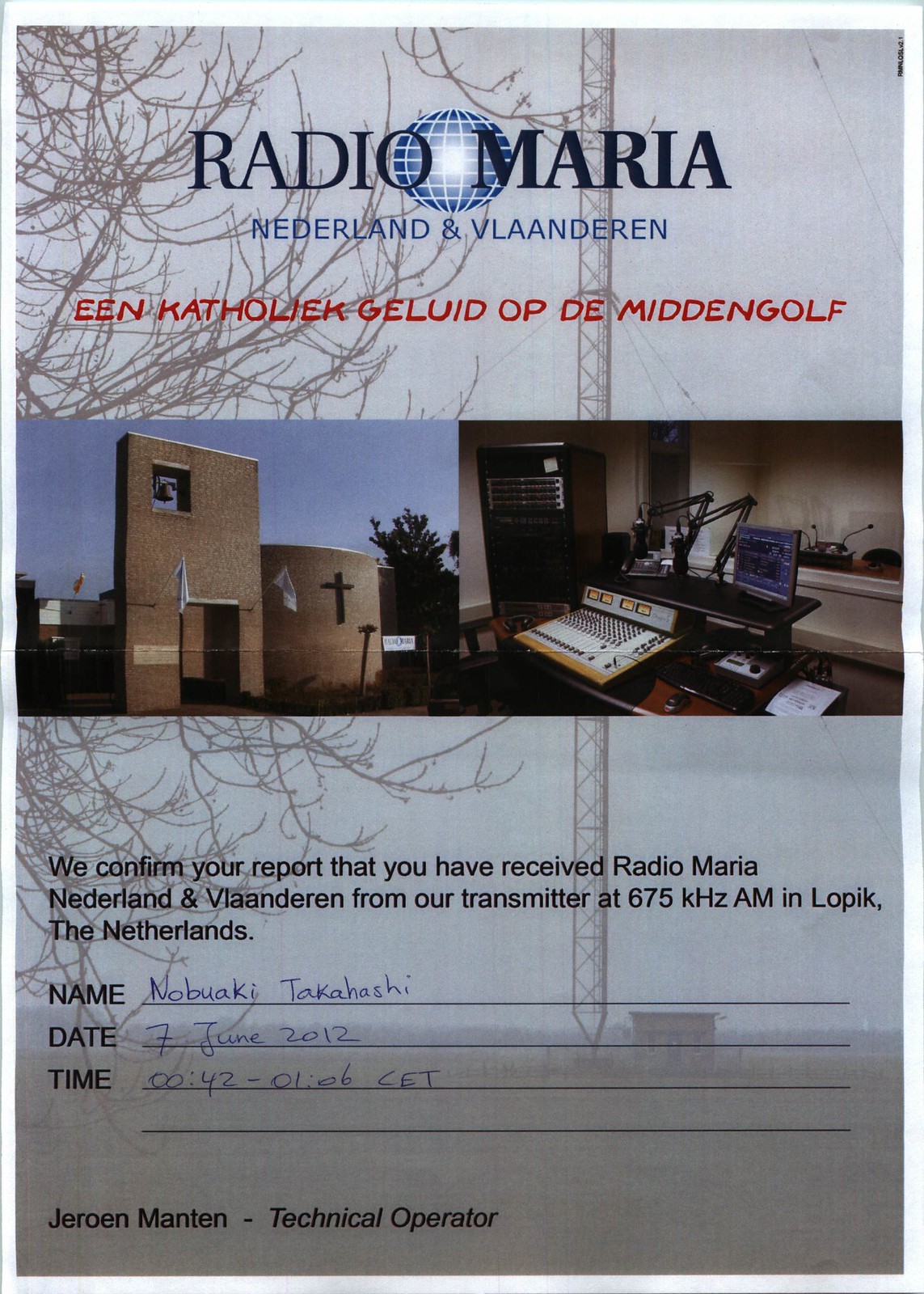This image features a tall, grayish flyer with the heading "Radio Maria, Netherlands and Vlaanderen" prominently displayed at the top. Underneath, there is red text that reads, "EEN Catholic Geluid op de Midden-Gulf." The flyer contains two photographs: one on the left of a church with a cross and two white flags, and another on the right showing the interior of a sound studio equipped with an audio board, microphones, a computer monitor, a black keyboard, and a mouse. The text below the photographs confirms the receipt of Radio Maria Netherlands and Vlaanderen from their transmitter at 675 kHz AM in Lopik, the Netherlands. The flyer also includes fields filled in by hand: "Name: Nabuaki Takahashi," "Date: 7th June 2012," and "Time: 42 minutes to one or 42 minutes past one." At the bottom, it is signed by "Jeroen Manten, Technical Operator."